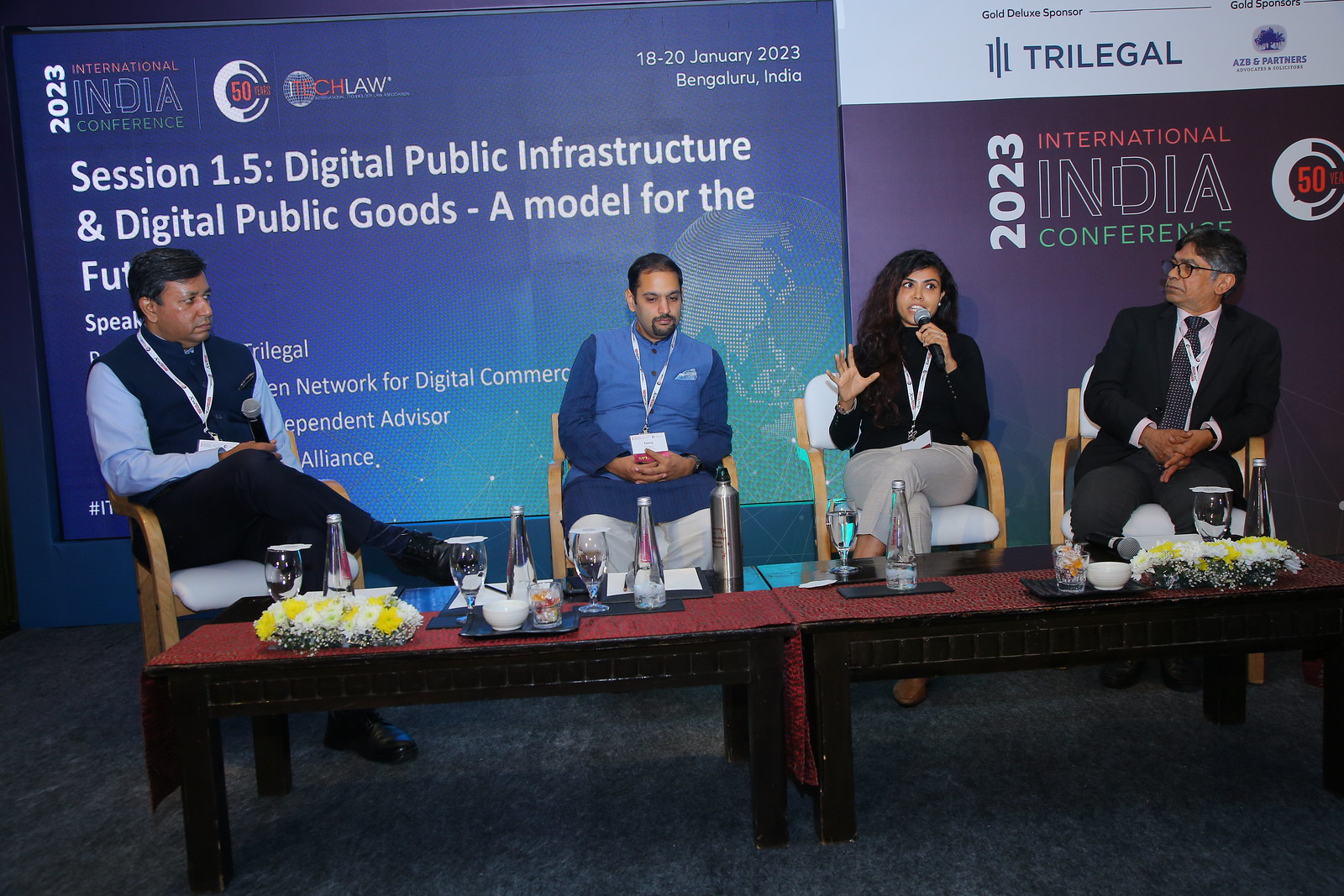The image depicts a panel of four people seated at a conference or presentation, detailed as the "2023 International India Conference" with the specific session titled "Session 1.5: Digital Public Infrastructure and Digital Public Goods - A Model for the Future." The background showcases a large blue banner with white text detailing the conference and session information, along with a secondary banner on the right side that is white and purple, featuring the sponsor "Trilegal" in blue letters. The panel consists of three men and one woman, each sitting in brown wooden-framed armchairs with white seat and back cushions. The woman, positioned third from the left, is actively speaking into a microphone with a silver ball on its end, her mouth open as she addresses the audience. In front of the panelists are two low, rectangular wooden coffee tables, pushed together to form a longer surface, and adorned with a matching red runner, creating the illusion of a continuous runner. The tables are decorated with multiple bottles, wine glasses, and floral arrangements featuring white flowers with yellow accents. Each panelist has water bottles placed in their individual areas for convenience.